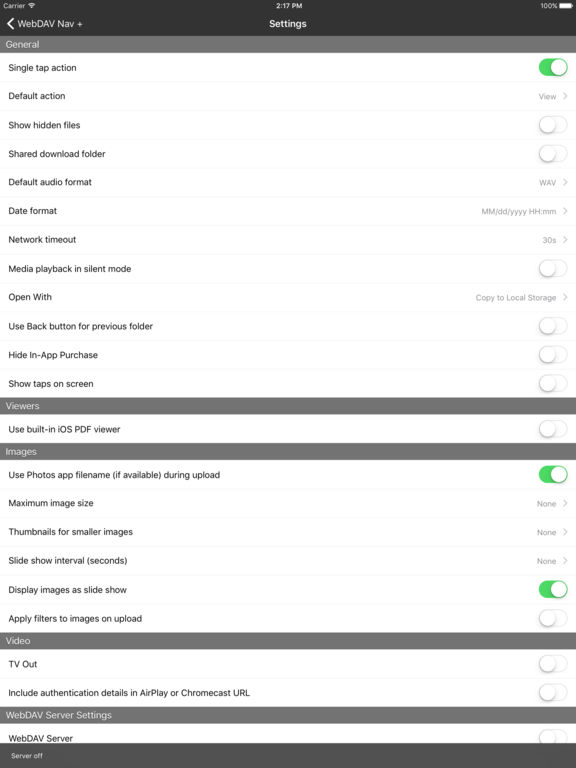### WebDAV Navigation Settings Page
The following is the detailed layout and status of the various settings on the WebDAV navigation settings page:

- **Background and Text:** The page has a plain white background with black text for readability.
  
- **Navigation and Sections:**
  - On the left side, there is a section labeled **"General"** in white text.
  
- **Settings:**
  - **Single Tap Action:** This option is switched on, indicated by a green slider button.
  - **Default Action Options:** Includes "View," "Show Hidden Files," and "Share." None of these options are currently selected.
  - **Auto Format:** The default setting is WAV.
  - **Date Format:** Configured to display as double digits for day and month, and four digits for the year.
  - **Network Timeout:** Set to 30 seconds.
  - **Media Playback in Silent Mode:** This option is turned off.
  - **Copy to Local Storage:** An option is present but not detailed in the status.
  - **Use Back Button for Previous Folder:** This setting is not selected.
  - **Hide In-App Purchases:** Not selected.
  - **Show Tabs on Screen:** Not selected.

- **Viewers Section:** Indicated by a gray bar.
  - **Use Built-in iOS:** Not selected.
  - **Use Photo App for Filename:** Selected.
  - **Display Images:** Selected.
  - **TV Out:** Not selected.
  - **Include Authentication:** Not selected.

This comprehensive description captures both the visual layout and the functional status of each setting on the WebDAV navigation settings page, providing a clear and detailed overview.